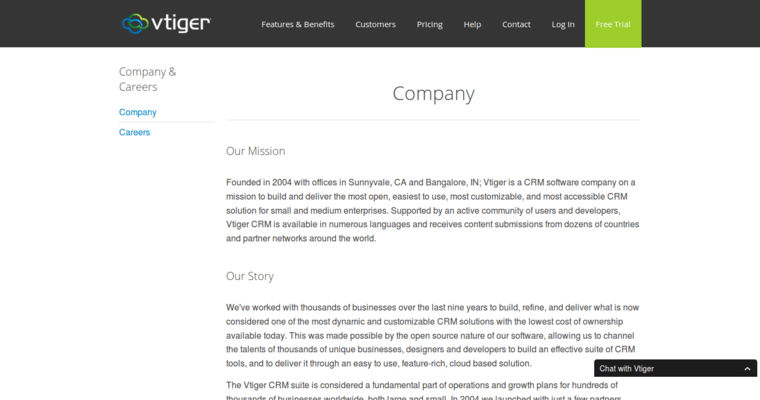In this screenshot, we are presented with a webpage from the company Vtiger. The top section features a black header displaying the company name "Vtiger" alongside their logo, which consists of an interlocked blue and green ring. To the right of the logo, the header contains navigation options in white text: "Features and Benefits," "Customers," "Pricing," "Help," "Contact," "Login," and an eye-catching "Free Trial" button highlighted in green.

On the left side, there is a panel labeled "Company" and "Careers." Beneath this, in blue text, the options "Company" and "Careers" are reiterated. Dominating the center of the page is a large heading in purple text that reads "Company." Below this heading, the subheading "Our Mission" introduces a detailed mission statement. The statement explains that Vtiger, founded in 2004 with offices in Sunnyvale, California, and Bangalore, Indiana, is a CRM software company dedicated to creating and providing the most user-friendly, customizable, and accessible CRM solutions for small and medium enterprises. This mission is supported by an active community of users and developers.